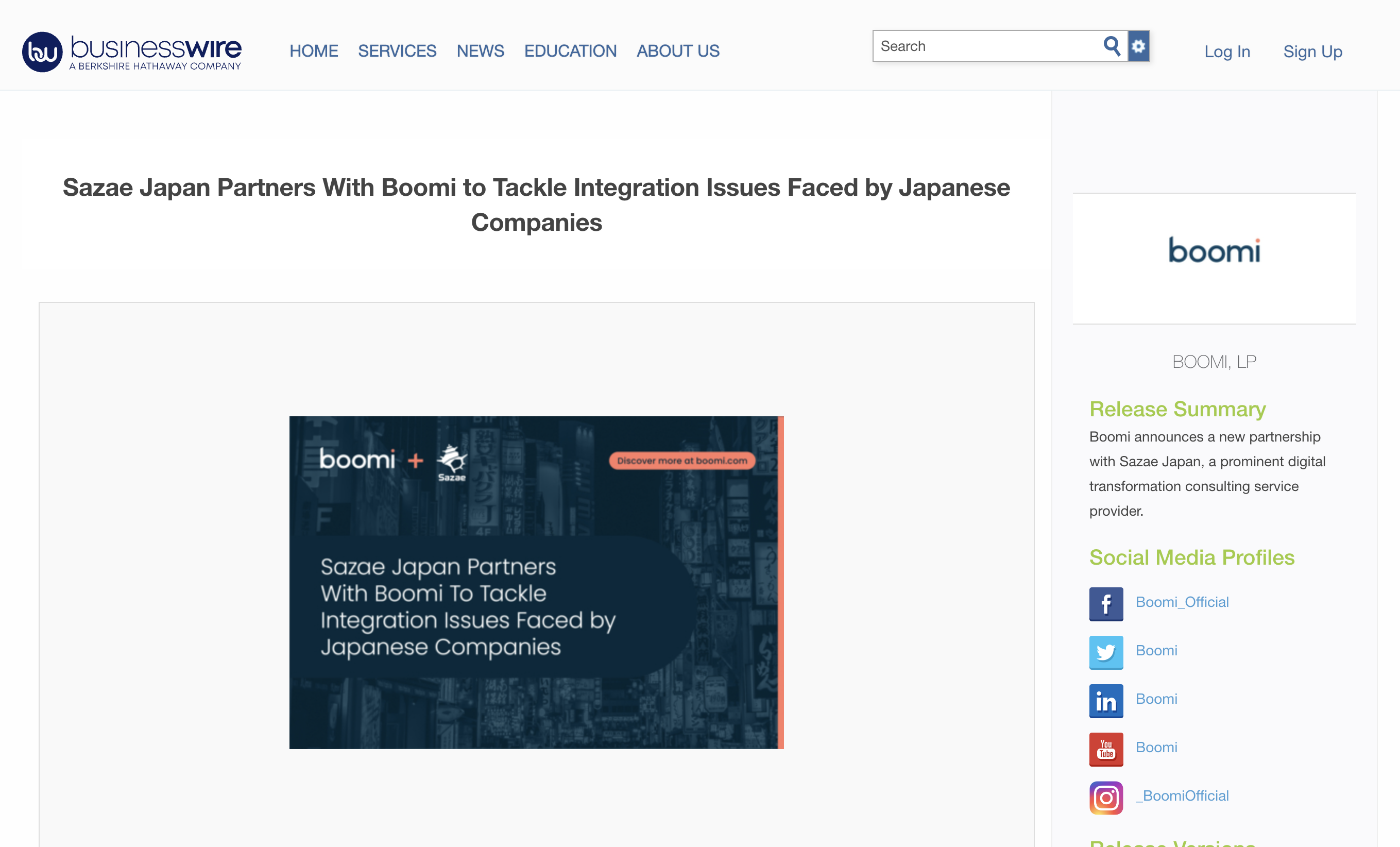**Caption:**

The top-left corner of the image features a blue banner with the text "BAU1W" and "Business Buyer, a Berkshire Hathaway Company." Below, there are navigation options labeled "Home," "Services," "News," "Education," "Advice," and "Search." Adjacent to this banner, black text announces, "Japan partners with Boomi to tackle innovation issues faced by Japanese companies." 

A prominent Boomi logo and text "Boomi+" are displayed against a red shell-like background. The caption also includes a call to action: "Discover more at Boomi.com." The central text reiterates Japan's partnership with Boomi to address innovation challenges.

A green text section, formatted like a release summary, states: "Boomi announces a new partnership with Sase Japan, a prominent digital transformation consulting service provider." Accompanying this, lime green text highlights Boomi's social media profiles, including Twitter (@Boomi), LinkedIn (Boomi), YouTube (Boomi), and Instagram (@Boomi_Official).

The overall background of the image is white, giving a clean and professional look to the detailed announcement of the strategic collaboration.